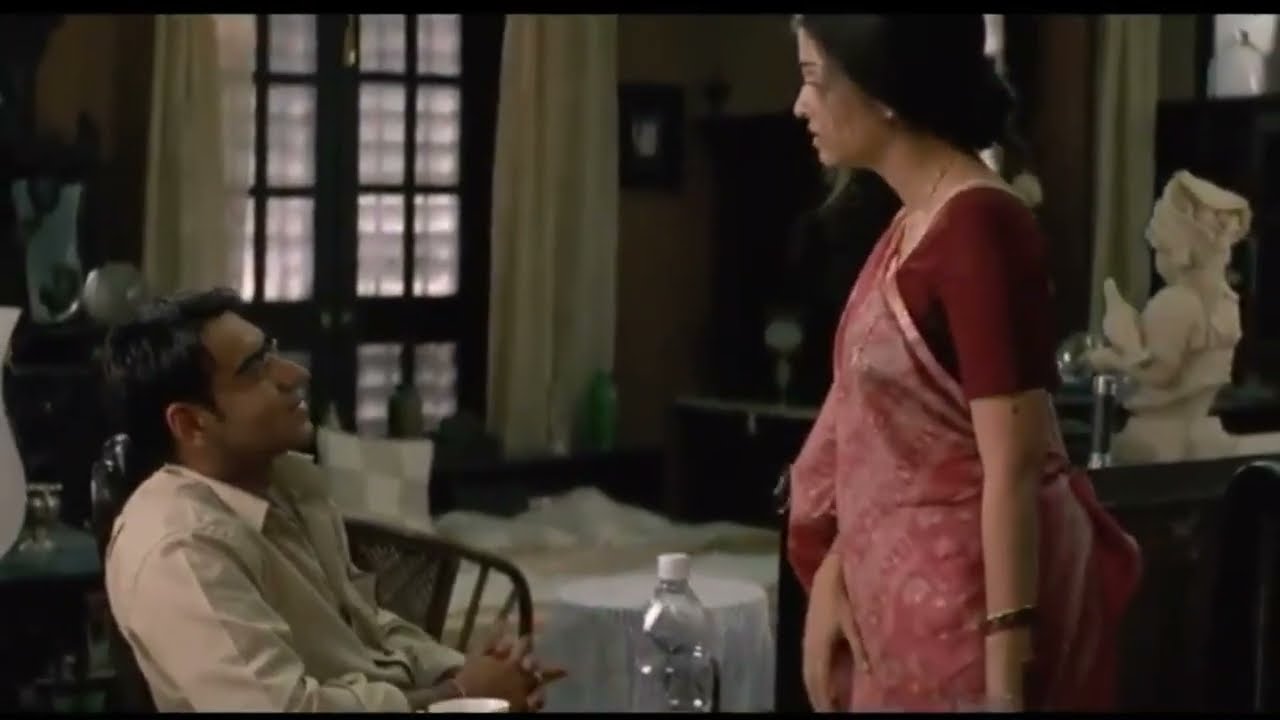The movie still depicts an intense scene between two individuals, likely of South Asian descent, engaging in a deep and possibly emotional conversation. The visually striking composition features a man with short black hair and darker skin sitting sideways in a dark chair, visible from the waist up. He is wearing a meticulously ironed white button-up shirt with the top two buttons undone and has his hands and fingers intertwined on his lap. His glasses reflect the dim lighting of the room as he gazes upward towards a woman standing to his right. 

The woman standing opposite him gazes down, her posture conveying a sense of serious engagement. She has her dark hair tied back in a bun and lighter skin compared to the man. She dons a striking red short-sleeved shirt complemented by a red shawl draped elegantly over her shoulders. Her outfit's richness is accentuated by earrings and a bracelet on her left hand. Positioned between them on the table is a clear plastic water bottle with a white cap, suggesting an ongoing or paused dialogue. 

The setting appears to be an indoor dining room with dim lighting, characterized by double doors with light curtains, a hint of a secondary table with a white tablecloth, and what seems to be a statue of a child with a bird on her arm in the background. Both figures appear to be deeply engrossed in their interaction, suggesting a moment of significant emotional weight or discussion.